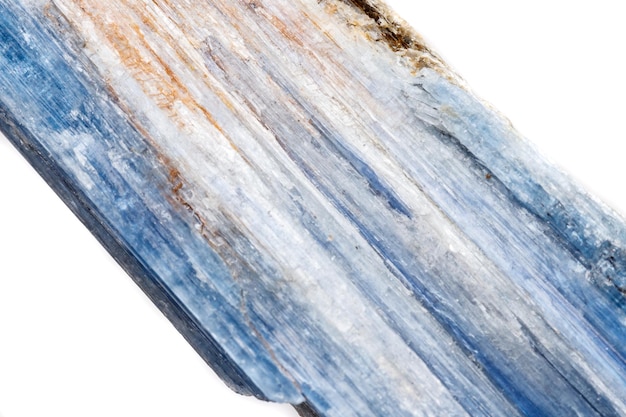The image depicts a mineral stone with a rough surface, displaying a prominent diagonally-oriented pattern. The stone transitions through multiple layers and shades, predominantly featuring an icy blue color mixed with streaks of white, light beige, gray, and brown. The left side base of the stone is distinctly blue, transitioning upwards through various hues, while the top right side shows a hint of brown. The mineral gives an impression akin to a shard of blue crystal, with a frosty and winter-like appearance, set against a white background that enhances its intricate and layered structure. The stone, somewhat rectangular in shape, appears scanned or magnified for detailed inspection, revealing its complex natural beauty.